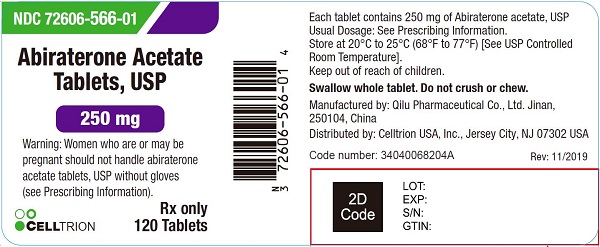Here is a detailed and cleaned-up descriptive caption for the image:

---

The label for Abiraterone Acetate Tablets, USP 250 mg is prominently displayed, with detailed information printed across various sections. In the upper left corner, a green rectangle features the label "NDC 72606-566-01" followed by a small purple stripe to its right. Centrally positioned on the label is a UPC barcode. Below the medication name and dosage, a cautionary note reads: "Warning: Women who are or may be pregnant should not handle Abiraterone Acetate Tabs, USP, without gloves. See prescribing information."

In the bottom left, the Celltron name and logo are clearly visible, along with the notation "Rx only" and "120 tablets." Moving towards the right, the manufacturing details are listed: "Manufactured by Quilly Pharmaceutical Co., LTD, Xinjiang, 250104, China. Distributed by Celltron, USA, Inc., Jersey City, New Jersey, 07302, USA."

Highlighted in the lower right part of the label is a red triangle enclosing a black box that says "2D code". Adjacent to this, the label provides fields for "Lot," "Expiration," "Serial Number (SN)," and "GTIN."

---

This version is structured to guide the reader’s eye through different parts of the label systematically, ensuring all important details are clearly conveyed.